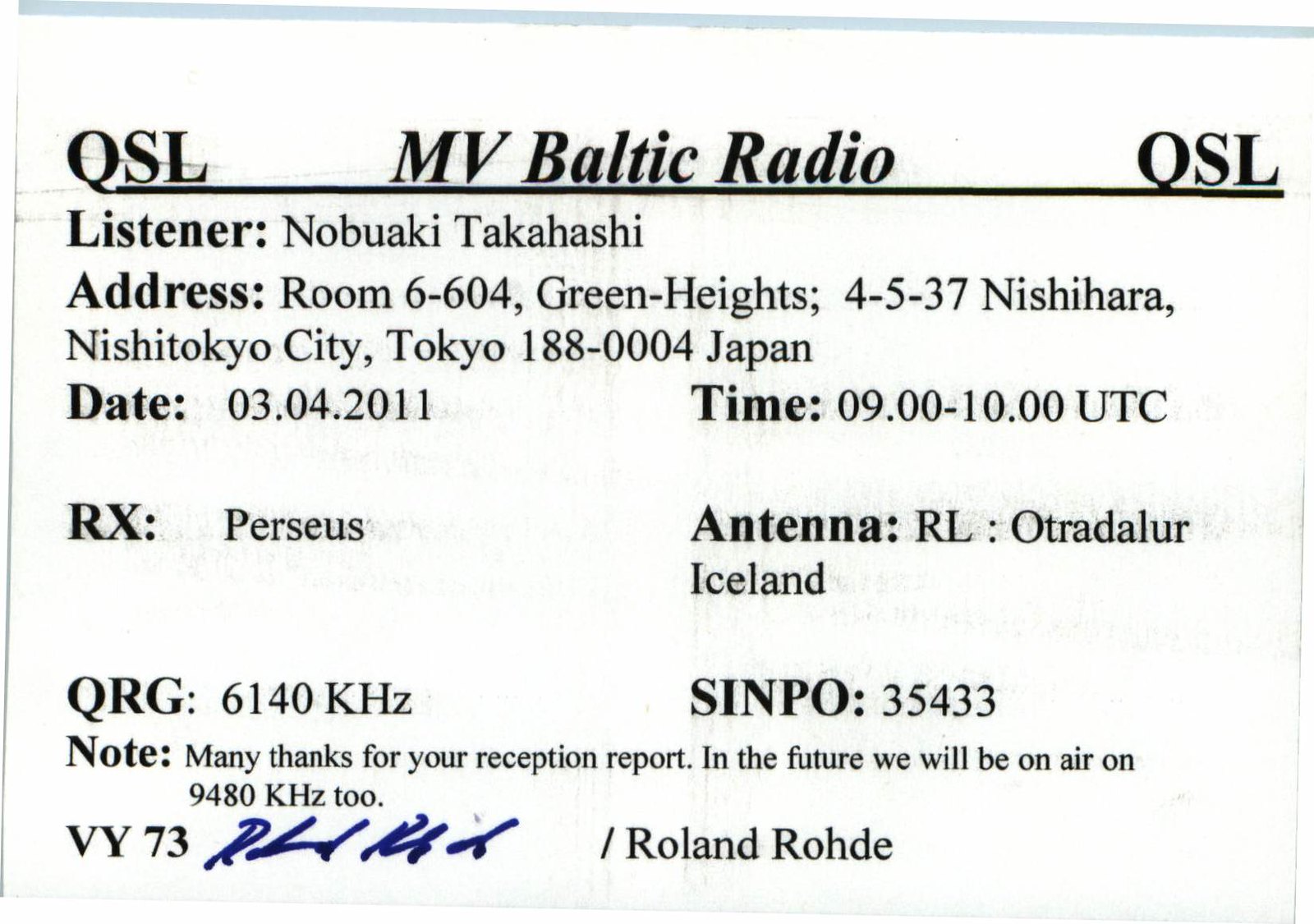The image displays a detailed report card-like document set against a white background with black lettering. Prominently, "QSL" appears in large letters both at the top left and right, with "MV Baltic Radio" centered between them, all underlined. Below this header, it designates a "Listener," Nobuaki Takahashi, followed by their address: Room 604, Green Heights, 455-37 Nishihara, Nishi-Tokyo City, Tokyo 188-0004, Japan. Subsequent entries list the date as March 4, 2011, and the time of reception. Fields labeled "RX" and "Antenna" indicate the receiver used was "Perseus" and the antenna was located in Otradalur, Iceland, respectively. Another section notes a frequency of 6140 kHz with a SINPO code of 35433. An additional message at the bottom expresses gratitude for the listener's reception report and mentions a future broadcast frequency of 9480 kHz. A dark blue signature by Roland Rohde accompanies this note.